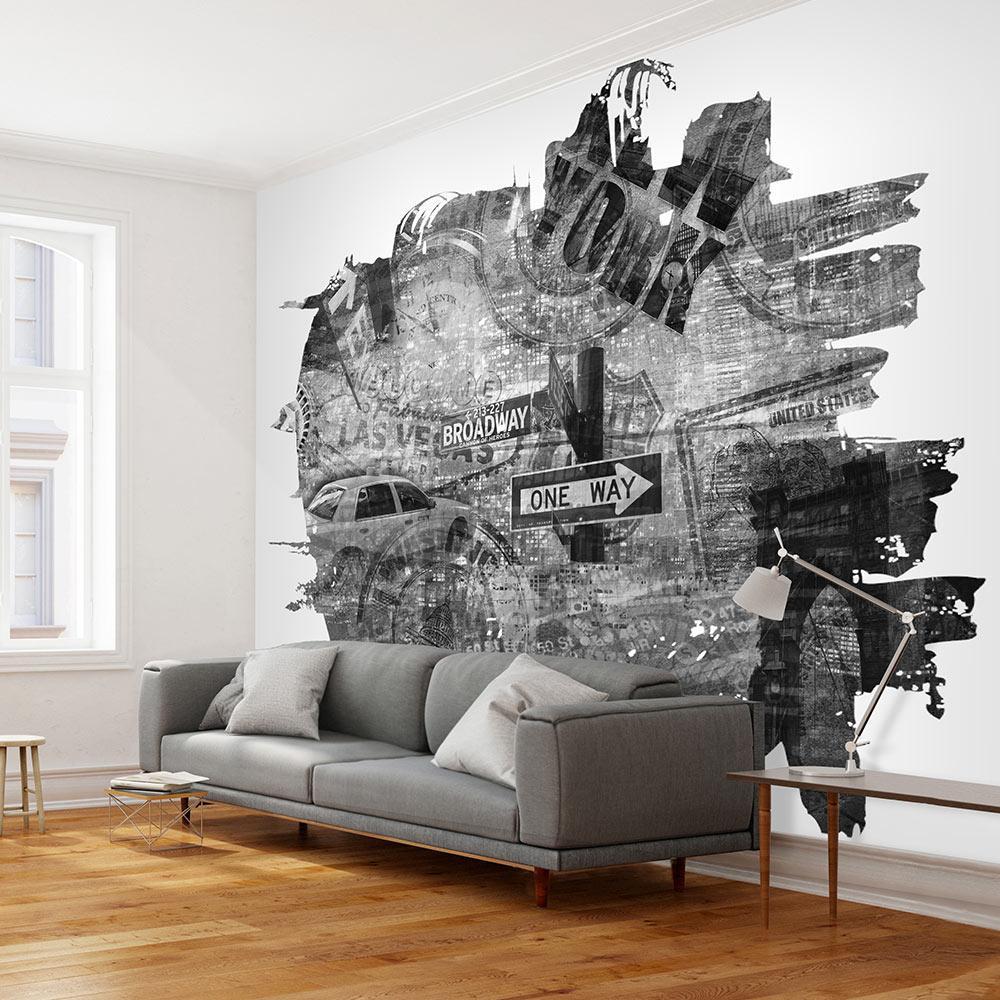The image showcases a living room in what appears to be an apartment, with a focus on one central white wall adorned with a large, intricate black-and-white mural. The mural incorporates various elements of American city life, such as iconic landmarks and signage. Notably, it features a Broadway sign, the words "New York" and "Fabulous Las Vegas," a one-way street sign, and a taxi cab, blending together in an abstract, variegated pattern as if applied with a paint roller. In the scene, a gray fabric couch with two pillows is positioned against this main wall. The room itself is minimally furnished, featuring a wooden floor, a side table with a lamp to the right of the couch, and a couple of stools, one of which holds a newspaper. A window on the adjacent left wall allows natural light to filter into the space, contributing to the overall simplicity and modern aesthetic of the room.